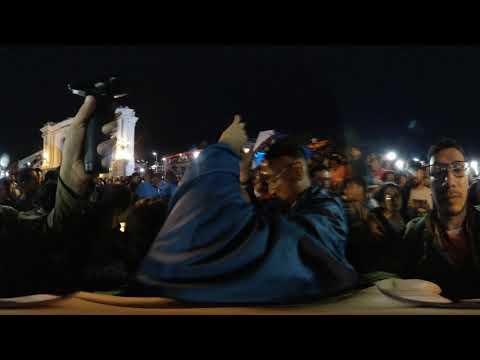The image is a nighttime panoramic photograph showcasing a dense outdoor gathering. The composition features a black border at the top and bottom, indicative of the image being stitched together from three different photos. At the forefront on the right side, an Asian man wearing glasses stares directly at the camera. Central to the image is a man in a blue jacket with a faint hint of blue hair, looking downward and slightly to the left. Just to his left, another individual holds up a black, small device, possibly an electric razor or toothbrush. The background is teeming with numerous people, many holding up camera phones that emit light, creating a captivating scene. The left section of the image shows a hand holding an object, in front of a lit two-story white building, and merges seamlessly into the central and right sections filled with bustling activity and lighted structures, all under a dark, starlit sky. This detailed night scene is rendered in a photographic representational style, capturing the realism and vibrancy of the event.